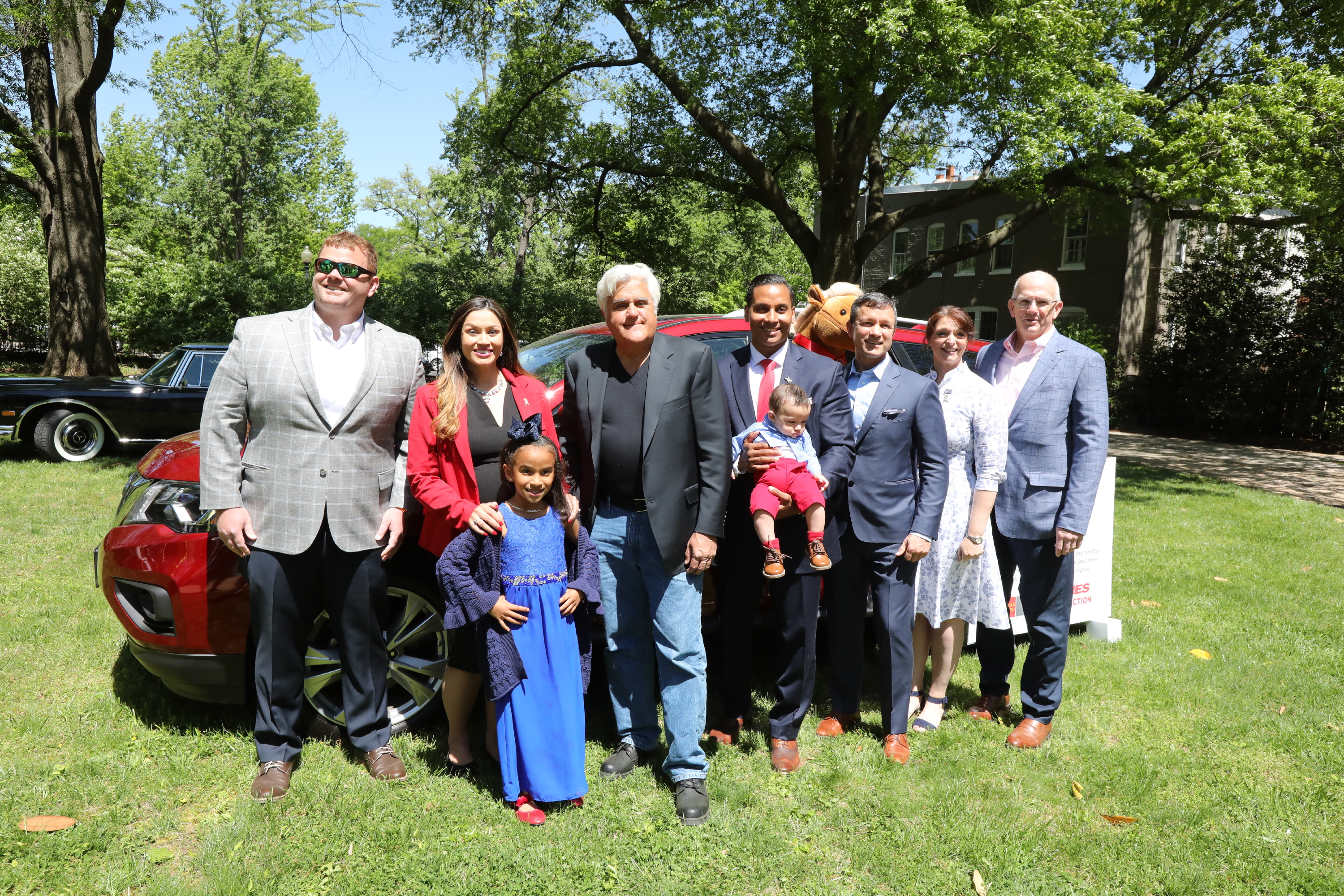This photograph captures Jay Leno, the famous comedian and talk show host, standing in the middle of a group of around nine or ten people of various ages. The group is positioned in front of a red SUV, which is partially obscured by them. Jay Leno, in a black sport coat over a tight black V-neck t-shirt, blue jeans, and black shoes, stands fourth from the left. To his left, there is a man, a woman, and a young girl, while to his right, there's a man holding a young child, another man, another woman, and an older gentleman on the far right. The scene appears to be outdoors on a grassy area with trees and a building visible in the background. A particularly intriguing detail is a very old Mercedes Pullman 500 Series SEL limo from the 60s behind the red SUV, which could pique Leno's interest due to his well-known passion for classic cars. The diverse group surrounding him seems to be a family, dressed in various attires, likely eager to pose with the celebrity in what appears to be either a backyard or a front yard.